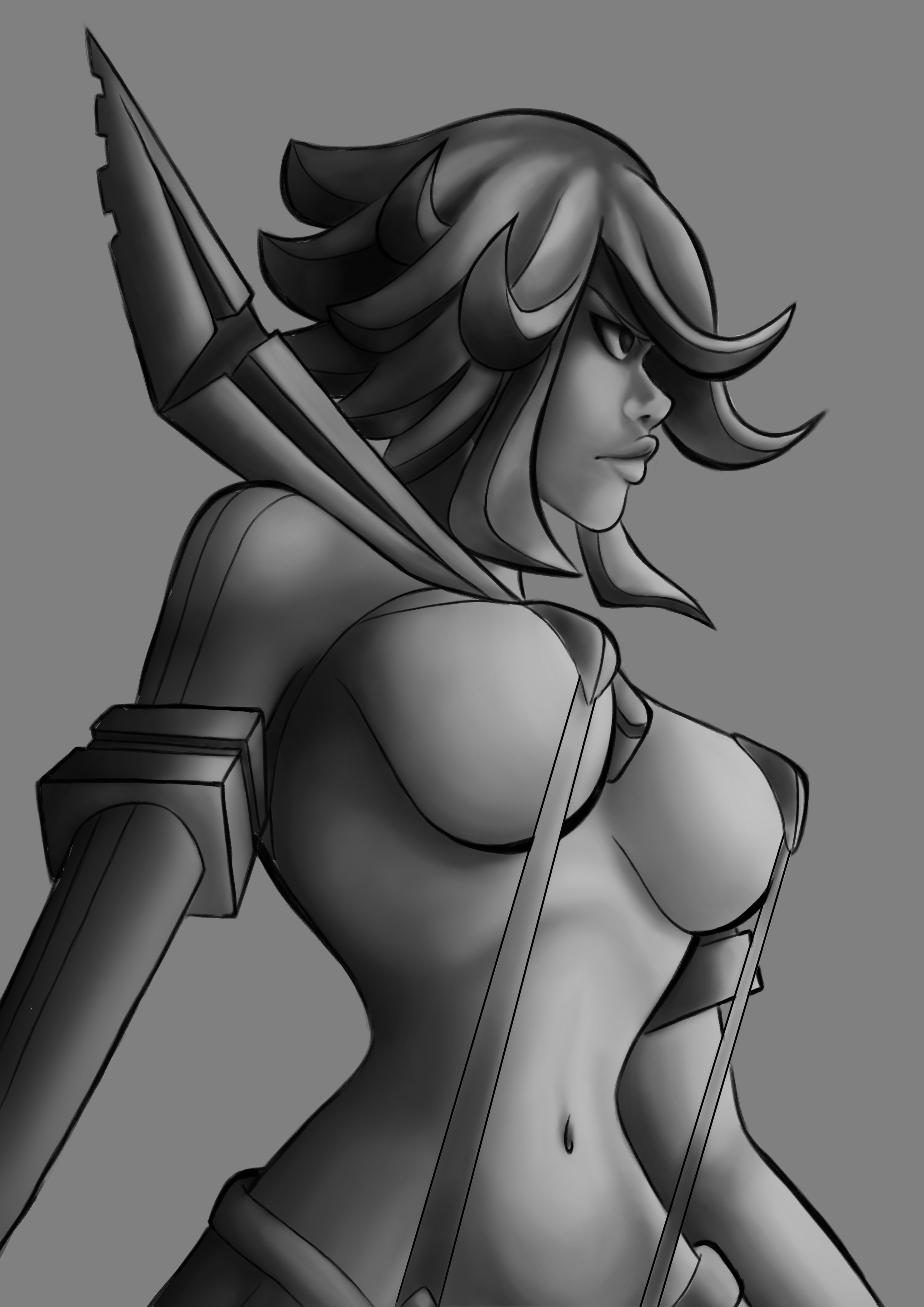This is a black and white, possibly digitally created illustration featuring a female avatar character with a distinctly cartoon or anime superhero aesthetic. The artwork is rectangular and entirely rendered in shades of black, white, and gray. The character, a woman with shoulder-length hair that waves upwards, is notably scantily clad, adorned only with a pair of pants and suspenders that barely cover her nipples. Her physique is highlighted by a very narrow waist. She stands slightly off-center, taking up most of the image, and gazes to the right side.

Her right arm appears to be mechanical, contrasting with her left arm. She wears square-shaped bracelets on her upper forearm and has an undefined object around her neck, which could be interpreted as a weapon or accessory. The background is a flat gray, further emphasizing her as the focal point of the piece. The overall style is reminiscent of an animated superhero comic cover, showcasing a blend of bold, feminine features and minimalist attire.